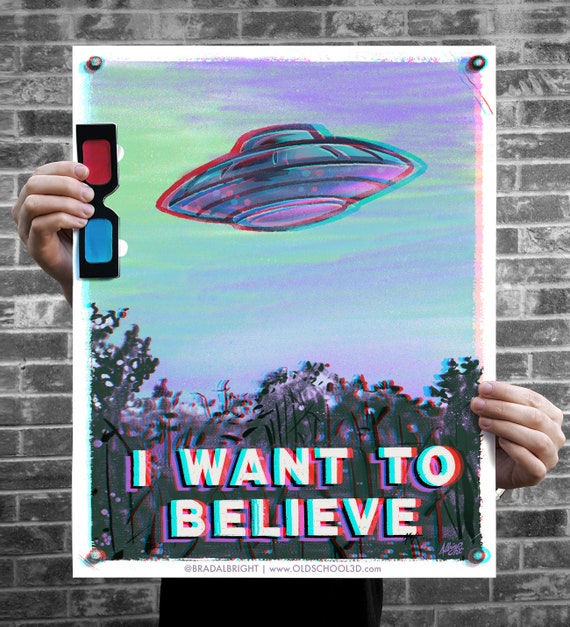The image depicts a person, mostly obscured except for their legs and hands, holding up a large poster against a brick wall. The poster displays a grayscale scene of a UFO hovering over a tree line, with the words "I WANT TO BELIEVE" prominently written in capital white letters across the bottom. The background sky behind the UFO contains hues of blue, green, and purple, giving it a unique 3D appearance. The grayscale elements contrast with this colorful sky. The person's left hand also holds a pair of black-framed red and blue 3D glasses in front of the poster. Along the very bottom white border of the poster, there's a smaller inscription that reads "AT BRADALBRIGHTWWOLD SCHOOL3DDOTCOM," referencing the artist and website.